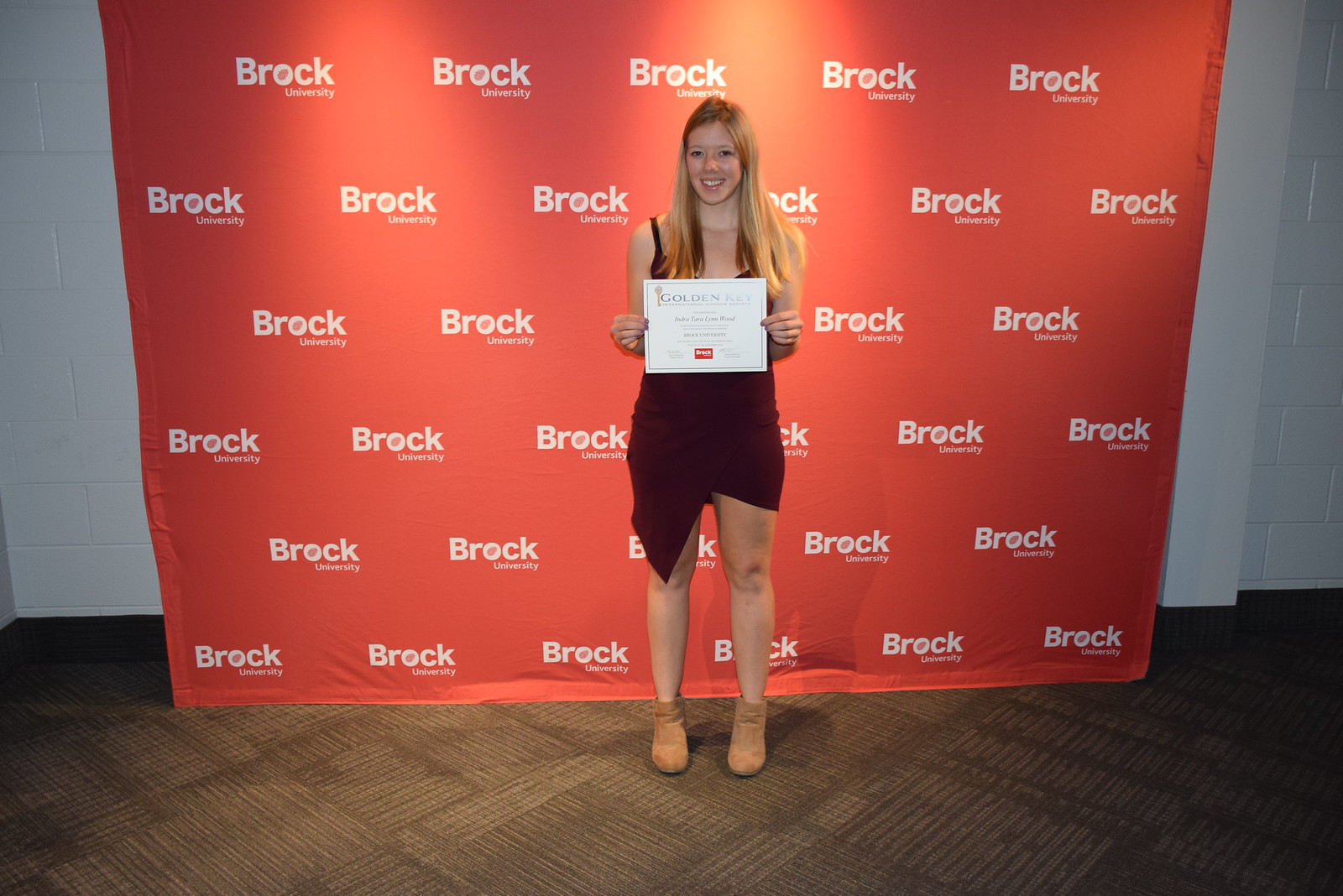A woman with rusty blonde hair stands on a brown tiled floor in front of a backdrop that repeatedly says "Brock University." The backdrop, designed for photo opportunities, is orange and smooth, positioned in front of a freshly painted white or off-white brick wall. She is wearing a burgundy, asymmetrical strapped dress with one side lower than the other, and tan shoes. She holds up an award certificate proudly, smiling brightly for the camera. The lighting is focused directly on her, highlighting her joyous expression.